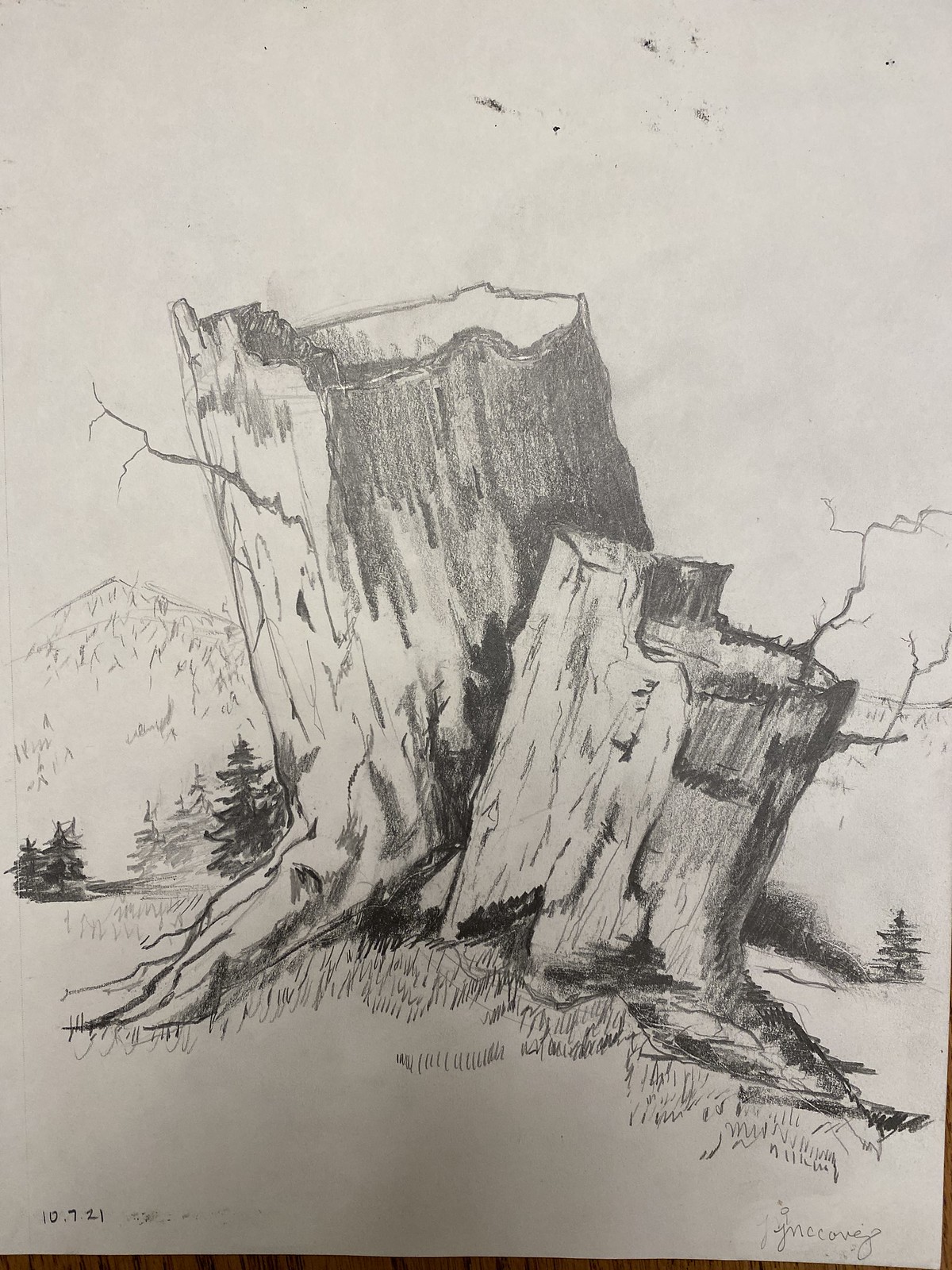This sketch depicts a cracked tree stump emerging from another tree, drawn meticulously with a 2B pencil. The artist employed horizontal shading and cross-hatching techniques to create texture and depth. The background features a variety of mountain shapes and outlines of trees, contributing to a sense of landscape. The date of creation, 09/10/21, is noted on the sketch, along with a faint, barely discernible signature in the bottom right corner. Despite the amateur style and the presence of smudges and fingerprints, the artwork conveys a rustic charm and attention to natural details.